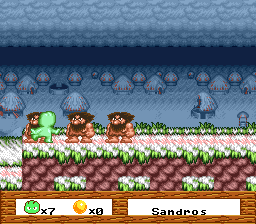A retro video game screenshot from a mid-to-late 1990s Nintendo game. The scene features three caveman-like characters and a green alien figure, either sitting or standing on pixelated brick platforms. In the background, a blue sky is punctuated with small, hut-like structures. Text overlays display "Sandro's" along with a score tally showing "7x" for the aliens and "0x" for golden balls. The image exudes nostalgic charm with its low-resolution graphics, typical of the era.